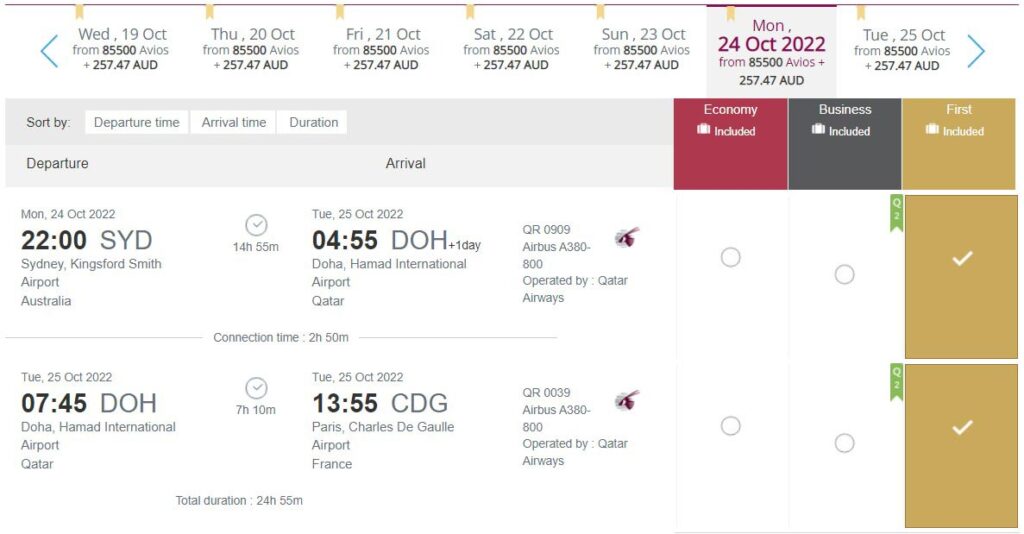This image, sourced from an airline website, shows a detailed flight selection process for various dates in October. At the top, the heading "Wednesday, October 19th" is prominently displayed along with the prices for different flights. For instance, the flight on October 19th is priced at 8,500 AVOs plus $257.47. The timeline extends through Thursday, Friday, Saturday, and Sunday, with the selected flight date highlighted in pink indicating "Monday, October 24th" in a larger, more noticeable light gray box. Additionally, a flight on "Tuesday, October 25th" is also mentioned with its respective pricing.

Below this date selection, the interface features a "Sort By" section on the left side with options to sort flights by "Departure Time," "Arrival Time," and "Duration." 

On the right, a selection of cabins is presented with maroon for "Economy Included," gray for "Business Included," and gold for "First Class," all accompanied by checkboxes.

Under the departure section, specific flight details include a departure time of 22:00 from Sydney and an arrival at Doha Hamad. Only the first column is selected, which appears to show another flight range from 07:45 to 13:55, again with a checkmark under "First Class." This detailed layout allows users to customize their flight preferences based on timing, duration, and class of service.